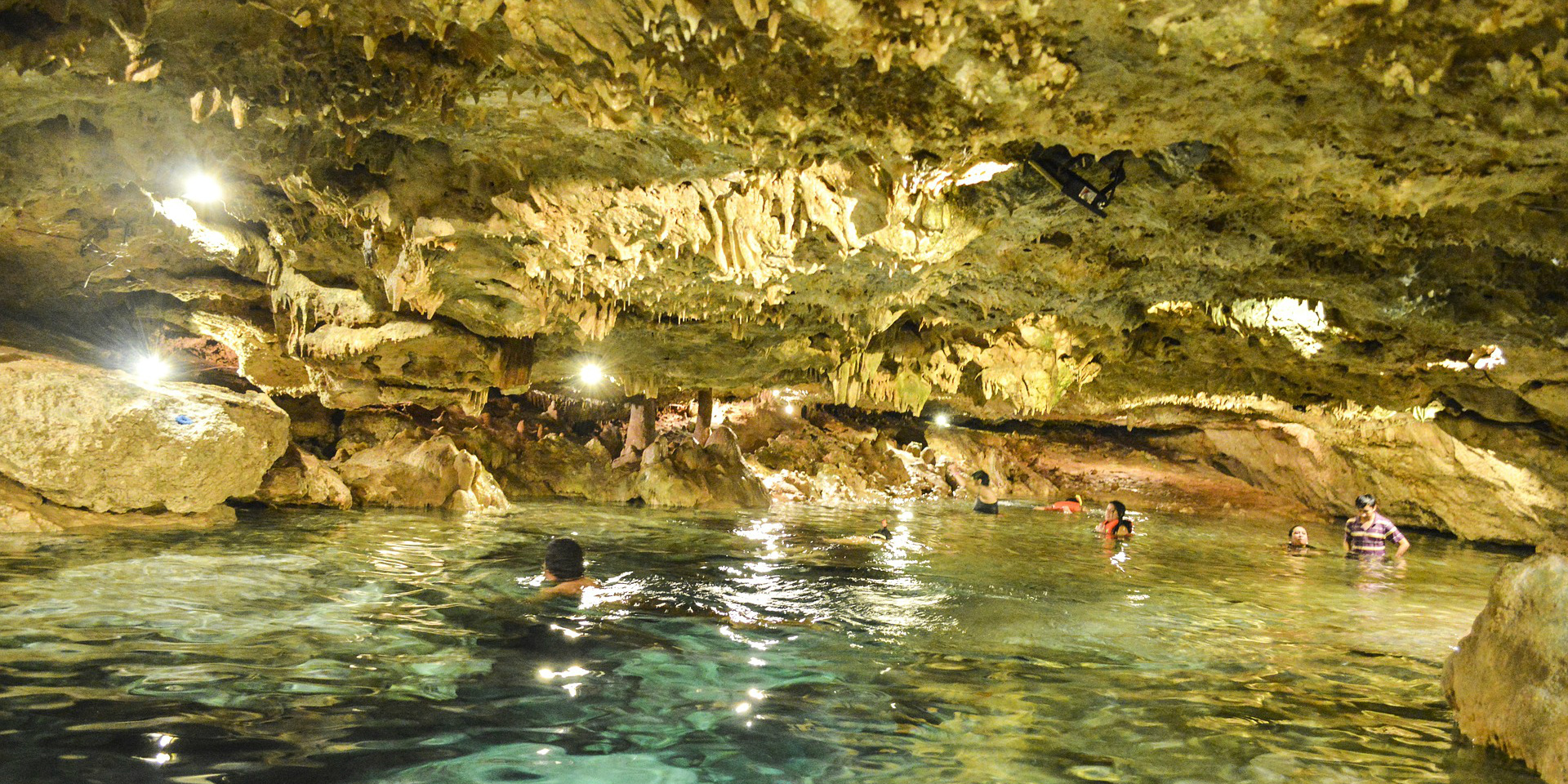The photograph captures a group of seven people swimming in an underground lake within a cave, possibly located near a bay. The cave, predominantly hued in brownish-beige with tints of green, is illuminated by light streaming through multiple holes in the ceiling, which may also be supplemented by artificial lighting equipment. Stalactites hang from the cave's ceiling, adding to the natural beauty of the scene. The clear water has a rocky bottom and appears dark green in color. The swimmers, including at least two children, two men, and two women, are in various swimming attire with some wearing life jackets. One man, identified by a black-and-white striped polo shirt, stands out on the right side of the image. The cave's serene atmosphere is enhanced by the calm water, shallow enough for people to stand in.